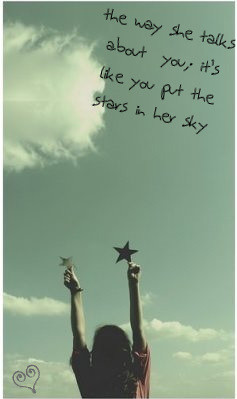The poster features a woman with long hair, standing in the bottom middle of the image, her arms extended straight up towards the sky. In each hand, she holds a star, likely gold or silver, though the image lacks vibrant colors and appears quite dull. She wears a light beige shirt. The sky is a light blue, with a prominent white cloud in the upper left corner and wispier clouds scattered towards the bottom. In the top right corner, in black, handwritten text, it reads: "The way she talks about you, it's like you put the stars in her sky." The bottom left corner of the poster displays a heart with tops that curl around each other instead of meeting in the middle.